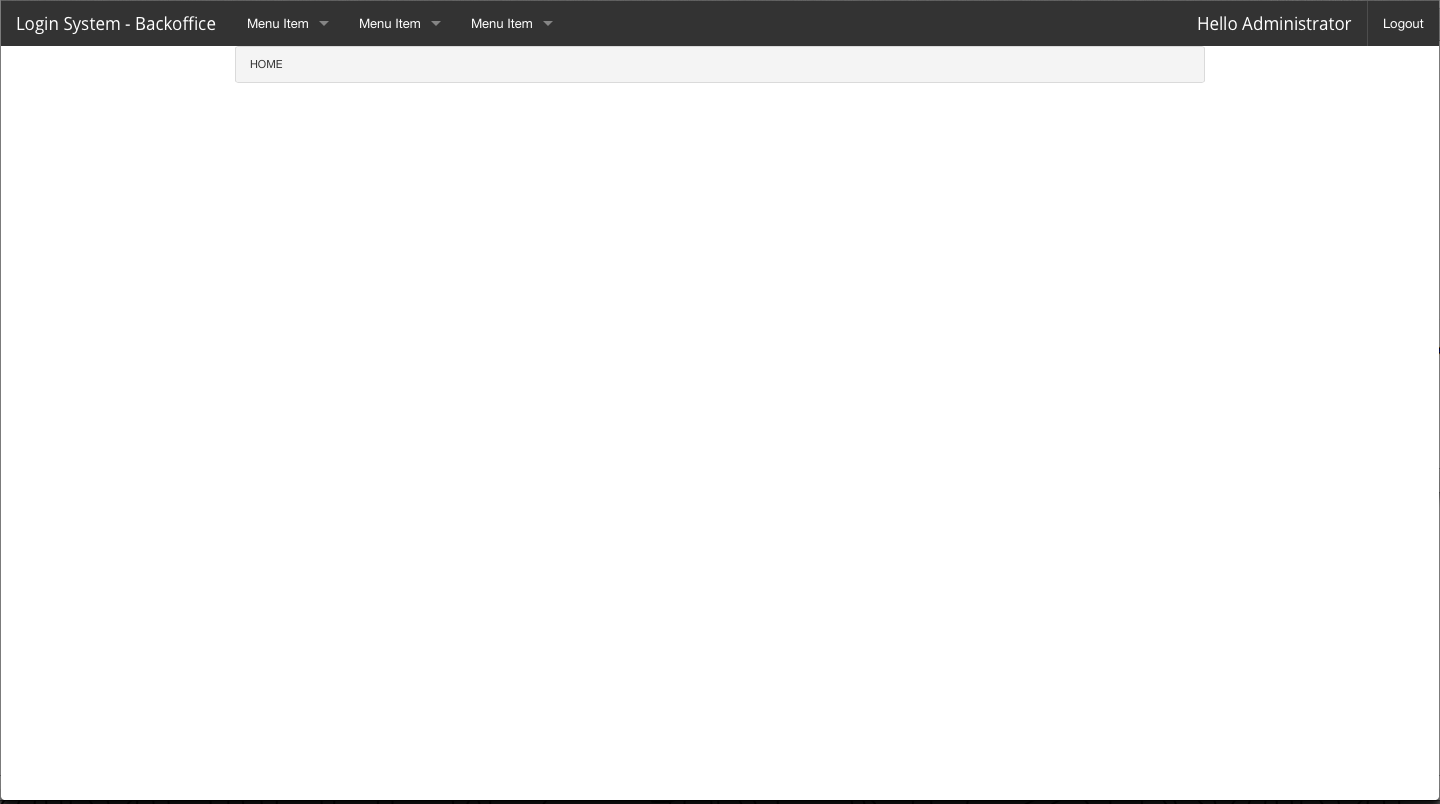The screenshot depicts a sparse computer interface, primarily blank with minimal content. At the very top, a black navigation bar spans across the screen. On the left side of this bar, the text "Login System-Backoffice" is displayed. Directly adjacent to this are three identical menu items labeled "Menu Item," each accompanied by a small downward arrow indicating a dropdown menu.

On the far right of the black bar, white text reads "Hello Administrator," followed by a vertical divider, and the "Log Out" option.

Beneath this navigation bar, the only visible content is the word "HOME" in all capital letters, located under the first menu item on the left. The remaining portion of the screen is entirely blank, aside from the faint outline of the page. This outline is delineated by light gray borders on the left and right sides, and a slightly thicker black border at the bottom.